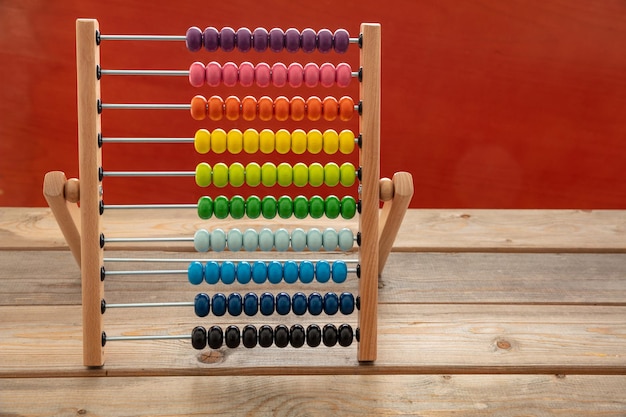A vibrant, child-friendly abacus is displayed prominently on a light wooden stand. The abacus features multiple rows of colorful, rounded beads. From top to bottom, the rows are arranged as follows: purple, pink, orange, yellow, light green, regular green, light blue, turquoise blue, navy blue, and black. All the beads are pushed to the right side of the abacus. The abacus sits atop a wooden plank table, and a red wall serves as a backdrop, enhancing the vivid colors of the beads. The beads are notably larger and rounder compared to traditional abacus beads, making them especially suitable for young children.